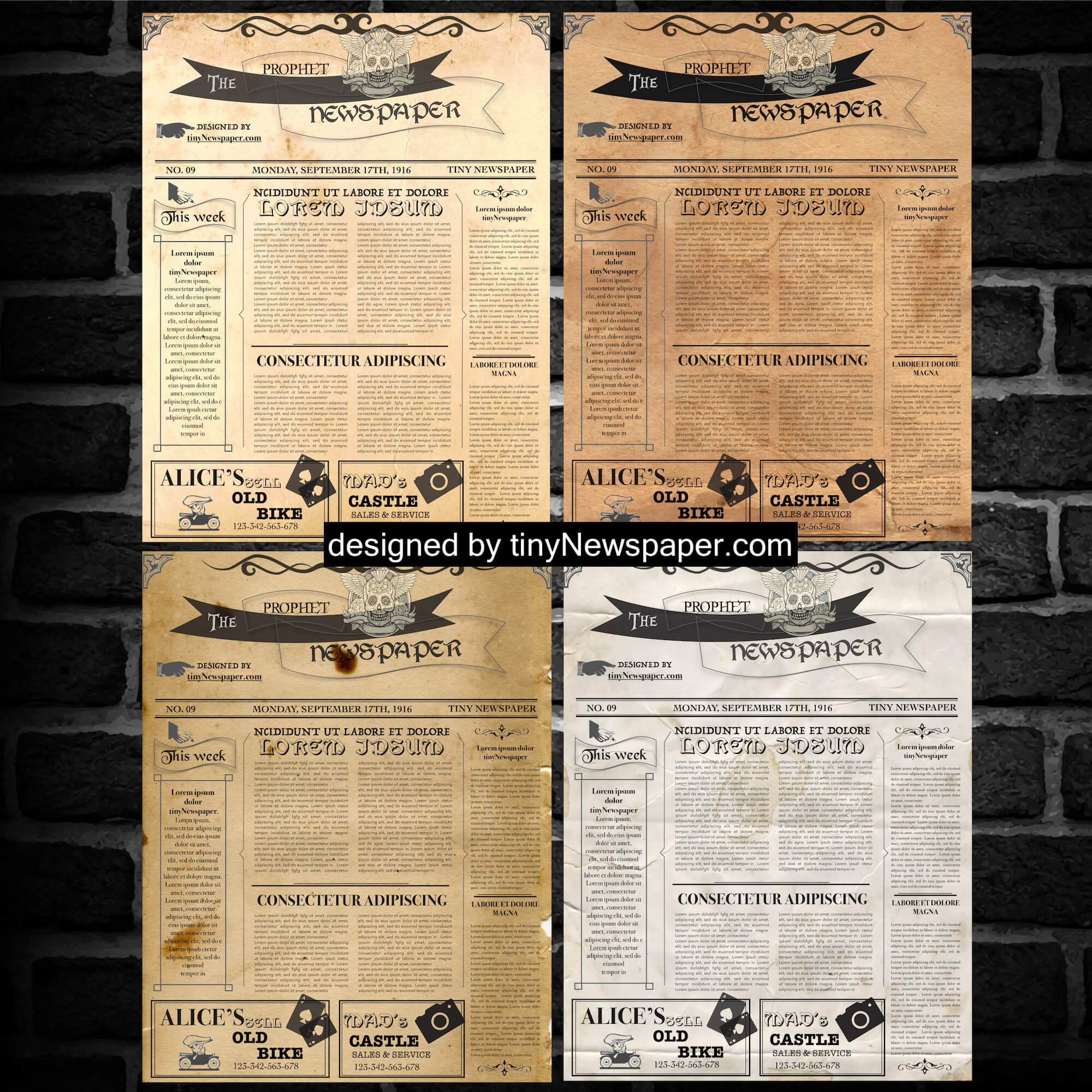The image features a square layout with a black and white brick wall background. Against this backdrop are four differently shaded newspaper prints arranged in a two-by-two grid. The newspapers are each dated Monday, September 17, 1916, and bear the title "The Prophet Newspaper." They vary in color, with one in a creamy shade, another brown, a third in a yellowish hue, and the last in black and white. Each paper includes similar content: an advertisement for Alice's old bike, articles, and a notable image of a skeleton. Centered within the image, over the newspapers, is the text "designed by tinynewspaper.com," highlighting the design variation. This arrangement likely showcases different design possibilities for the same edition of the newspaper.